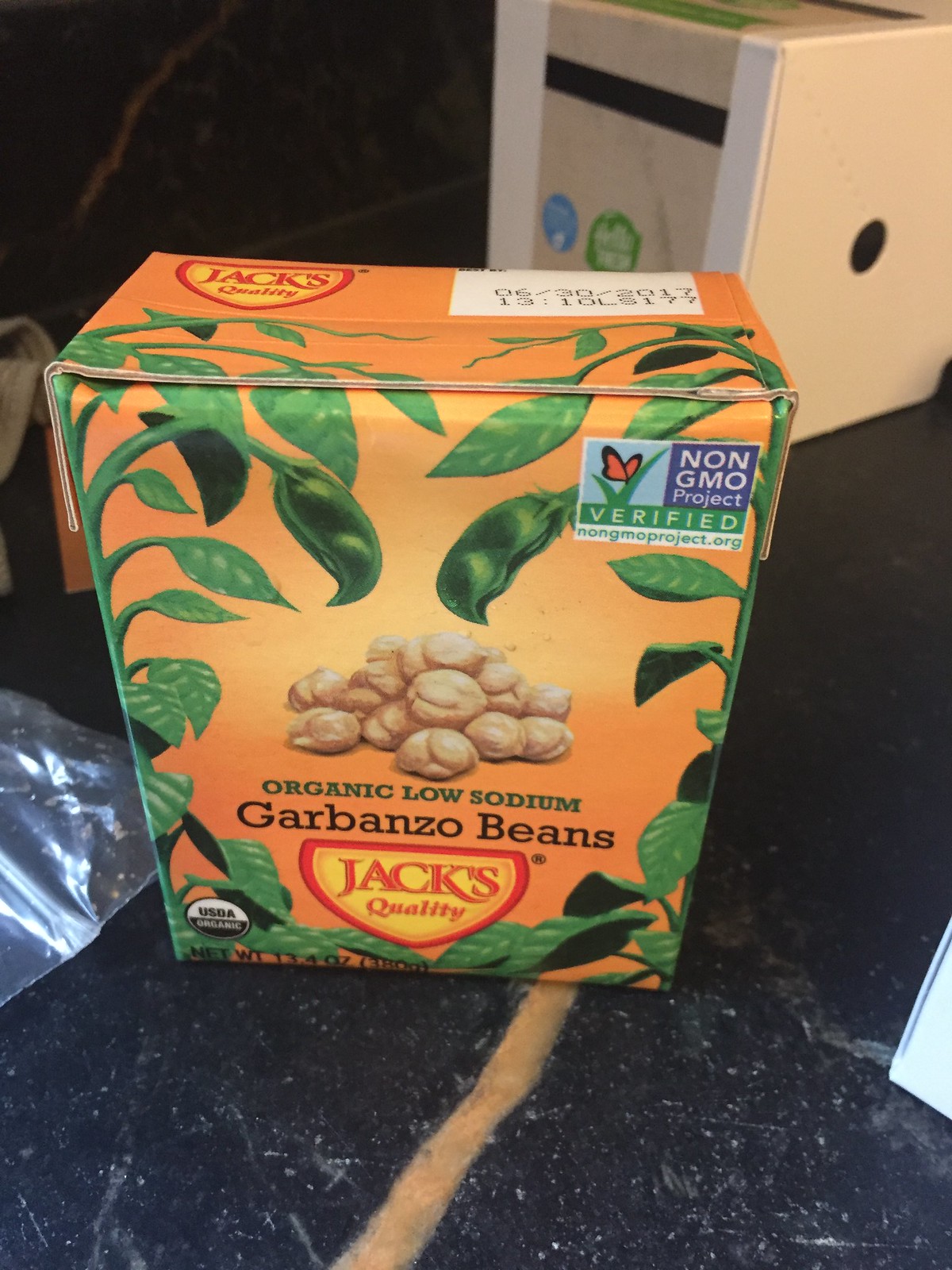The image displays an orange box featuring green leaves ornamenting the top left and right corners. In the center of the box is a heaping pile of garbanzo beans. The beans are labeled with "Organic Low Sodium Garbanzo Beans." Directly below this text is a yellow shield with a red border, emblazoned with the logo "Jax Quality." On the bottom left corner is the USDA Organic certification, while the top right corner showcases a square graphic with grass leaves and a butterfly, highlighting the Non-GMO Project verification, authenticated by nonmoproject.org. In the background, there is a white box with white bars along the left and right sides, and a black bar in the middle. The top and bottom segments of the box display a tan color.